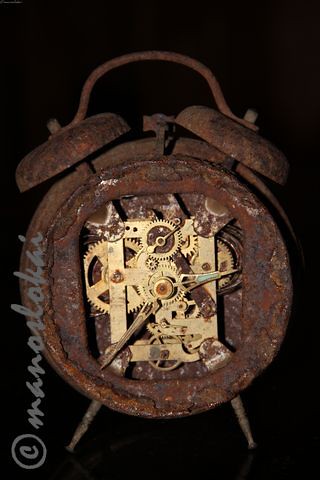This image showcases a rusted alarm clock, heavily corroded on its exterior to the point of near-total decay. Interestingly, the back of the clock is open, providing an unobstructed view of its intricate internal mechanisms. Despite the outer deterioration, the clock's interior remains pristine: the gears and components glimmer in stark, untarnished gold, creating a dramatic contrast with the rusted shell. Both the minute and hour hands are visible, hinting that the clock's timekeeping functions are intact. The extent of the exterior rust suggests prolonged exposure to harsh elements, possibly even submersion underwater for years, reminiscent of an artifact retrieved from a shipwreck. This juxtaposition of decayed exterior and immaculate interior offers a fascinating glimpse into the clock's resilience and mechanical intricacy, suggesting that despite its aged and weathered appearance, it may still be in working condition.